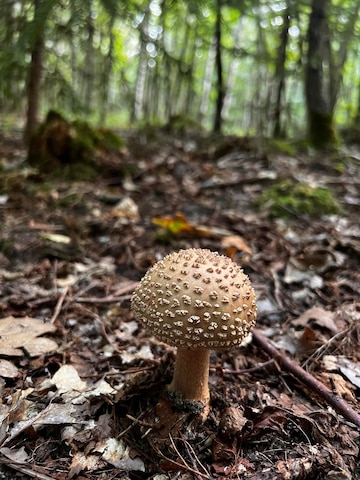In the foreground of a wooded forest, a single, tan mushroom with a thick, slightly darker stem stands prominently. The mushroom, appearing larger than it is, features a rounded cap adorned with numerous rough protrusions resembling a knobbly pattern. The ground around it is a rich, dark brown, covered in bark, dead leaves, pine straw, twigs, and other leaf litter, creating a mulchy texture. 

The sunlight, seemingly coming from the right-hand side and back, illuminates the scene, casting intricate shadows and highlighting the mushroom’s unique texture, which is smooth underneath. In the background, a quiet forest full of thin tree trunks, mostly brown with some white, such as birch trees, recedes into a blur of green foliage and light, contributing to a sense of depth and tranquility. Some of the trees bear green leaves, and there's a hint of green among the forest floor's otherwise brown palette. A moss-covered stump is visible among the blurred trees, adding to the woodland atmosphere. 

The high horizon line further emphasizes the focus on the mushroom, ensuring it dominates the lower half of the image while the softly lit and blurred trees fill the upper half. The overall effect is a serene and intimate forest scene, with the singular mushroom as the detailed and textured focal point amidst a natural backdrop.